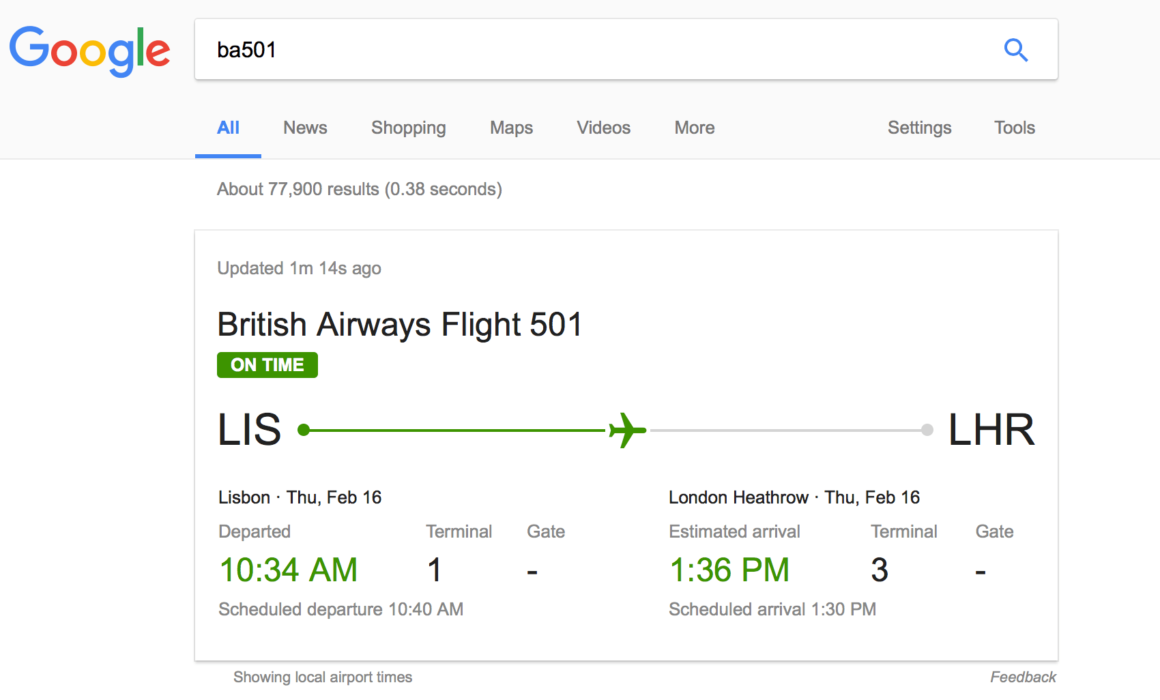This image is a cropped screenshot of a Google search for flight information. The search bar at the top displays "BA501", referring to British Airways Flight 501. The search results show a prominently displayed white box with "British Airways Flight 501" written in large text. Below that, a green box indicates the flight status as "on time."

In the center of the white box, the airport codes are displayed: "LIS" for Lisbon and "LHR" for London's Heathrow Airport. These codes are connected by a horizontal bar with a plane icon in the middle, illustrating the flight path.

On the bottom left of the box, the departure time and terminal information from Lisbon are shown. On the right side, the estimated arrival time at Heathrow Airport and the corresponding terminal are displayed. Additionally, in small grey text at the top left corner of the white box, the last update is noted as being "updated 1 minute 14 seconds ago." This detailed information was generated immediately after the user entered "BA501" into the search bar.